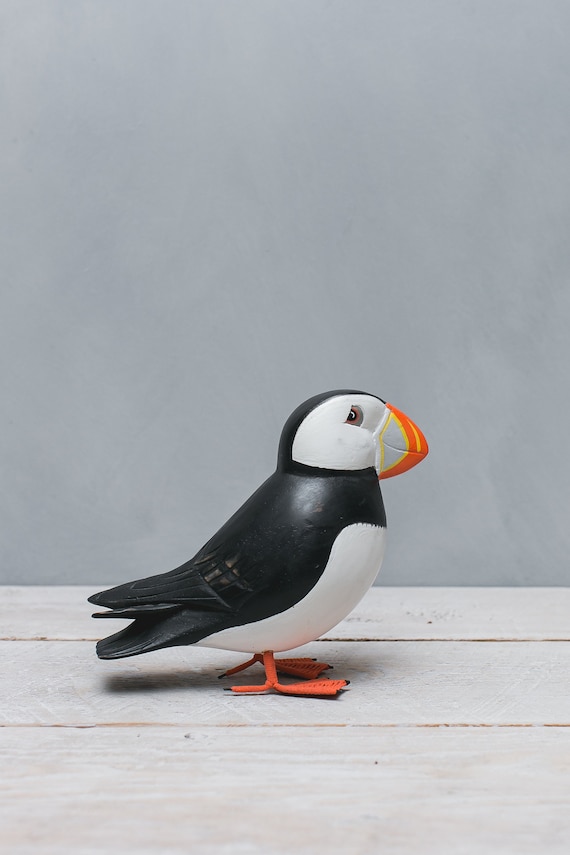The image is a detailed photograph of a carved puffin sculpture positioned in the lower center of the frame. The puffin stands on pale tan wooden planks with a rough finish, likely part of a floor or table, against a solid light gray wall. The puffin's head is predominantly white with a black stripe at the back, and it features distinct orange, yellow, and gray accents on its beak. Its eyes are deep-set, small, and black, surrounded by white. The puffin's wings are black, its belly is white, and its orange feet have black tips on the toes. The majority of the gray background is undisturbed, highlighting the puffin as the central focus. The sculpture, which appears to be made of plastic, looks lifelike yet is evidently inanimate. The absence of any other items or text in the photograph ensures that the viewer's attention remains on the detailed and colorful representation of the puffin.